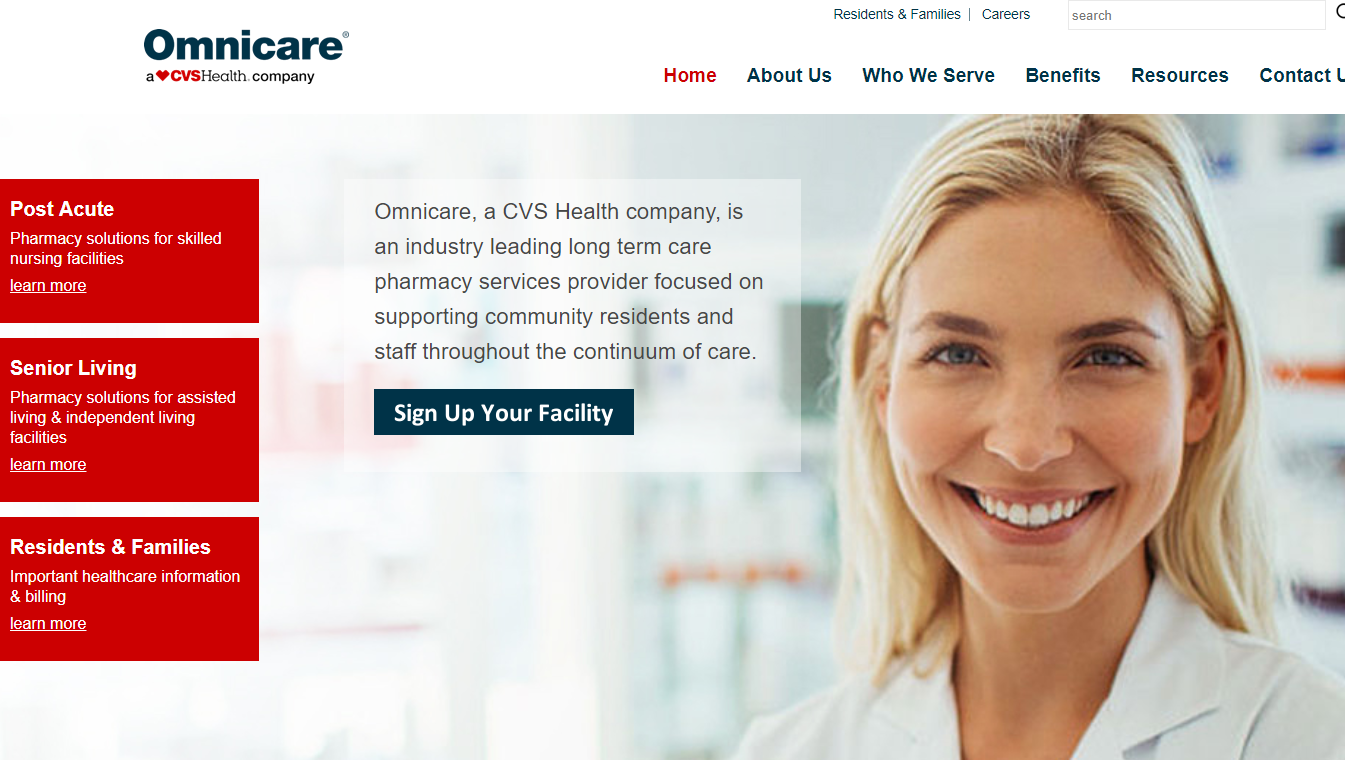This is a detailed screenshot of the Omnicare website, clearly designed for a CVS Health company. Dominating the right side of the image is a photograph of a young woman with blonde hair and blue eyes, centrally positioned to catch the eye.

In the upper left-hand corner is the Omnicare logo, proudly stating "a CVS Health company." The header at the top of the screenshot provides navigation options with phrases like "Residents and Families" and "Careers," alongside a search bar for easy access.

Highlighted in red letters at the top right, there is a prominent "Home" button. Alongside it are additional navigation links: "About Us," "Who We Serve," "Benefits," "Resources," and "Contact Us."

The left-hand side of the image features three red rectangles with white lettering, each providing service details. The first rectangle reads "Post-Acute," describing pharmacy solutions for skilled nursing facilities. The second rectangle says "Senior Living," which details pharmacy solutions for assisted living and independent living facilities. The third rectangle is labeled "Residents and Families," offering important healthcare information and billing details.

Positioned in the middle left, adjacent to the photograph, is another rectangle containing text about Omnicare. It reads: "Omnicare, a CVS Health company, is an industry-leading long-term care pharmacy services provider focused on supporting community residents and staff throughout the continuum of care."

There's also a call to action, "Sign up your facility," encouraging engagement.